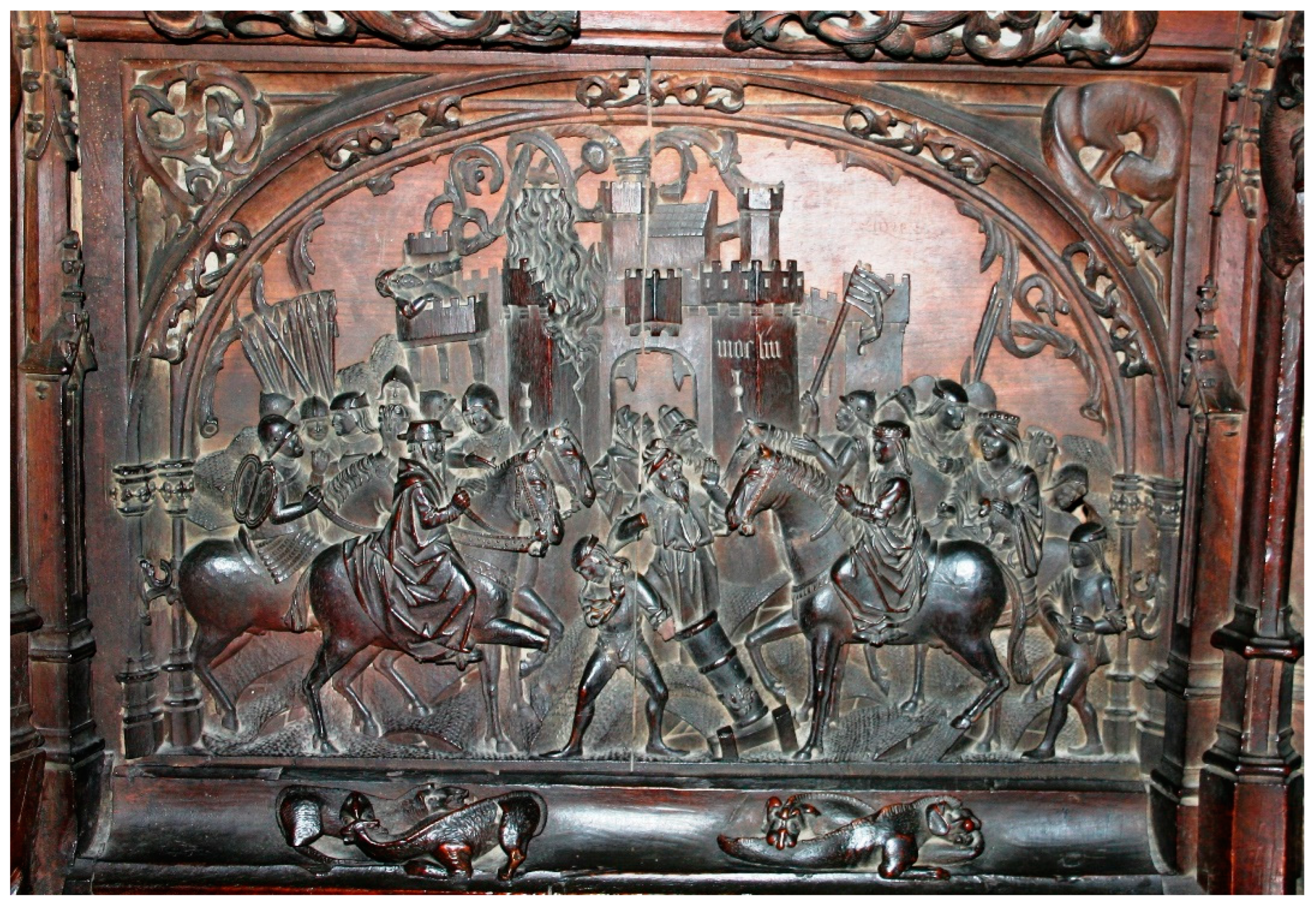This detailed wood carving, possibly a wood engraving darkened with age, adorns cabinet doors and depicts a dramatic medieval scene. The central focus is a grand castle in the background with its portcullis drawn up, indicative of an impending or active siege. In the foreground, two opposing factions are vividly portrayed: one consisting of kings and lords, and the other of religious figures including women dressed in crowns and robes, all on horseback engaging in battle. Flags are raised, illustrating the intense clash. Among the intricately carved figures, a character seems to operate a cannon aimed at the castle. Additionally, peculiar reptile-like creatures populate the bottom of the carving. The doors, colored in a reddish hue, contrast strikingly with the metallic design embellishments, overall providing a rich and immersive depiction of medieval warfare.